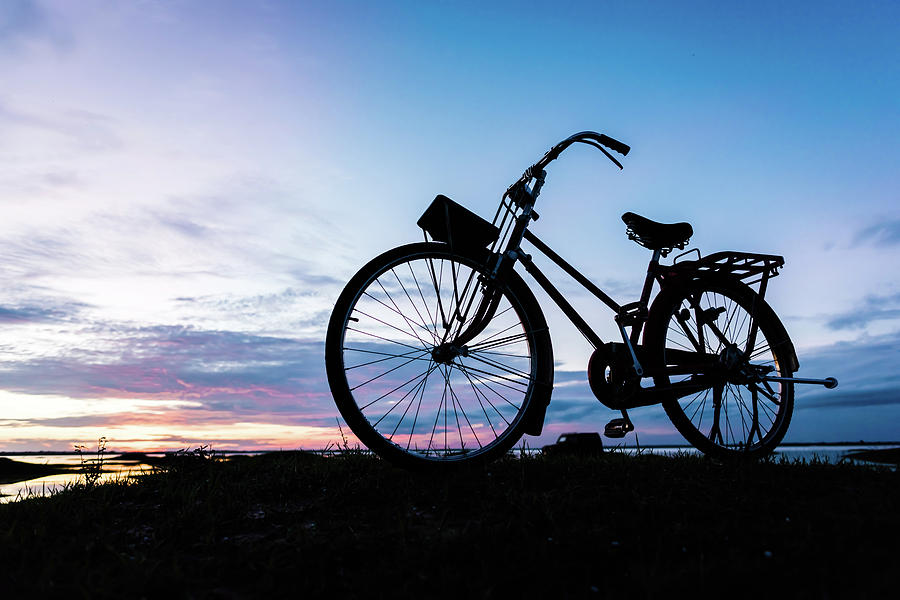The photograph captures a classic silhouette of an old-fashioned bicycle against a stunning sunset sky, hovering over a black grassy beach, possibly near an ocean. The horizon bisects the scene roughly at the lower quarter, where the ocean meets a sandy or grassy terrain. The bicycle, centrally placed towards the right, exhibits a plain frame with a luggage rack in the back and sweeping handlebars. An unusual feature is its numerous spokes, about twice as many as a standard bike's. The sky is a gradient, transitioning from a pinkish hue near the horizon to a deepening blue towards the top, interspersed with thin, wispy clouds. In the distant background, a vehicle can be discerned between the bike's tires, blurred but notably present. The overall ambiance is serene, with the setting sun casting dim light, allowing only the bike's silhouette to be prominent against the intricate twilight sky.